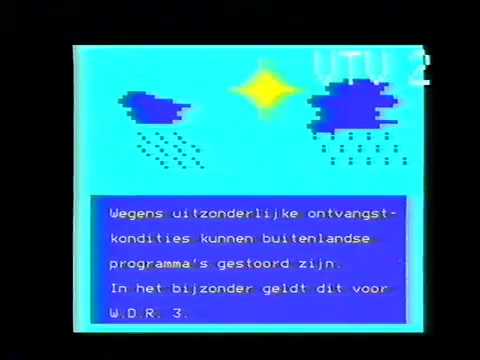This image features a photograph of a rectangular screen, likely from an old computer monitor or TV, showing a pixelated, 1980s-style video game interface. The screen is predominantly light blue, akin to a robin's egg or Tiffany blue, with a solid black border surrounding it. Prominently displayed on the screen are dark blue clouds, one on the left and a larger one on the right, both emitting precipitation—rain from the left cloud and more scattered, snow-like particles from the right. Centrally positioned between the clouds is a bright yellow, primitive-looking sun. The bottom of the screen contains a dark blue rectangular block featuring white text written in a foreign language, surrounded by a black background. The word "VTV2" appears in white letters at the top of the screen, enhancing the retro, pixelated aesthetic of the image. The overall layout suggests it is a snapshot of an old-fashioned video game with very basic, squared graphics.